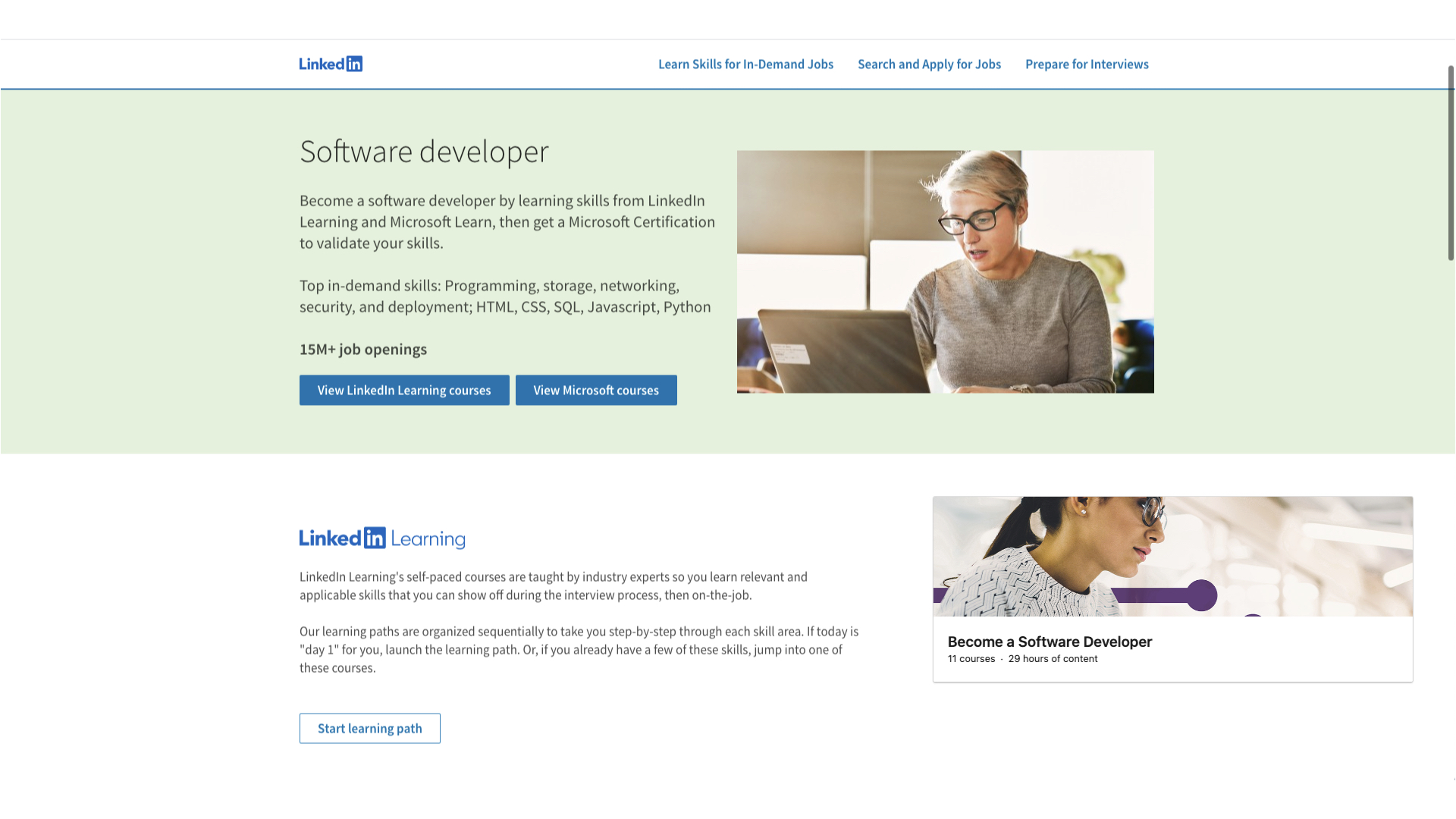**Detailed Caption:**

This image is a screenshot of a LinkedIn webpage dedicated to promoting courses for aspiring software developers. The LinkedIn logo is prominently displayed in the top left corner, while navigation links are positioned at the top right. These links include options such as "Learning Skills for In-Demand Jobs," "Search for and Apply to Jobs," and "Preparing for Interviews." 

The page features a headline in bold text: "Become a Software Developer." Below this headline, a description reads: "Learn skills from LinkedIn Learning and Microsoft Learn, then get a Microsoft certification to validate your skills." 

A list of top in-demand skills follows, enumerating essential proficiencies like Programming, Storage, Networking, Security, and Development. Specific languages and technologies such as HTML, CSS, SQL, JavaScript, and Python are also highlighted.

Two prominent blue buttons below this section offer further navigation options: "View LinkedIn Learning Courses" and "View Microsoft Courses." A note beneath these buttons states, "15 million+ job openings," underscoring the demand for software developers.

An image accompanying the text shows a person intently working on a laptop, representing a typical software development scenario.

The lower section of the screenshot provides a detailed description of LinkedIn Learning. It describes the platform's offerings as self-paced courses taught by industry experts, enabling learners to acquire relevant and applicable skills. The description emphasizes the sequential organization of learning paths and the flexibility they offer, which help learners showcase their skills during interview processes and in their subsequent jobs.